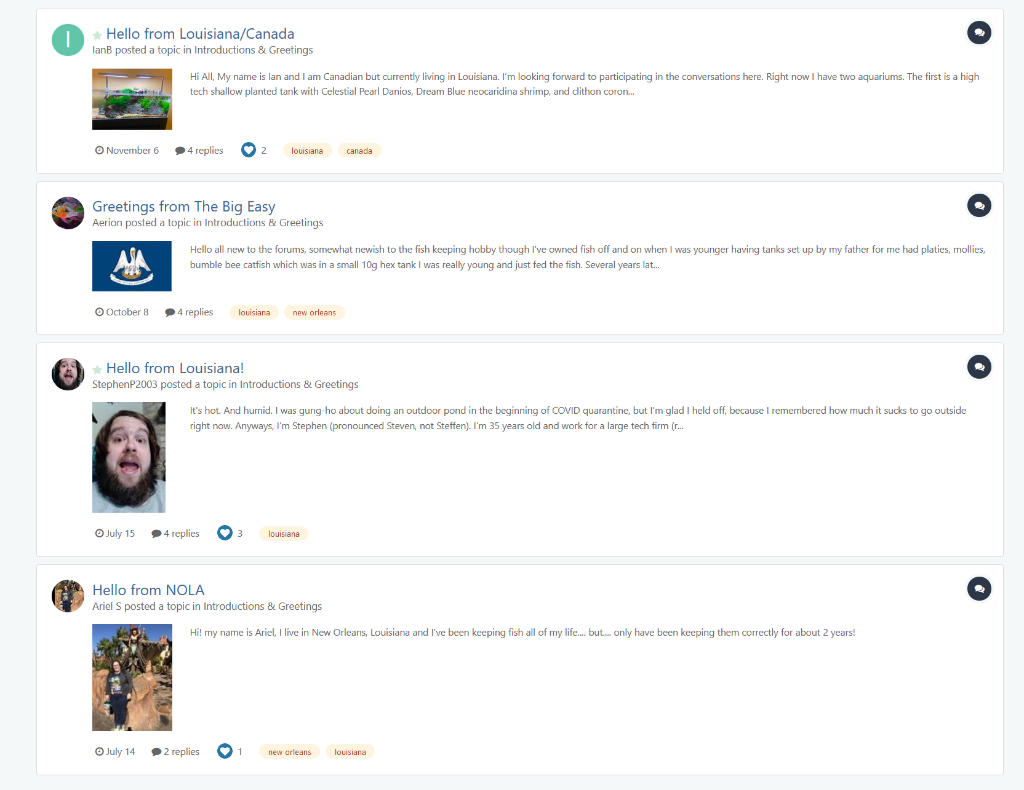### Landing Page Overview for Discussion Threads

---

This detailed depiction of the landing page showcases four discussion threads, each on a light grey background with white rectangular cards. Let's break down each thread:

1. **Thread One: "Hello from Louisiana/Canada"**
   - **Icon**: Green with a large white eye in the center.
   - **Header**: "Hello from Louisiana/Canada" in blue.
   - **User Info**: "IANB" in grey.
   - **Category**: "Introductions, Greetings".
   - **Content**:
     - Image on the bottom left: A photograph of what looks like a fish tank with a beige wall and greenery inside, illuminated by two overhead lights.
     - Post: "Hi all, my name is Ian, and I am Canadian but currently living in Louisiana. I'm looking forward to participating in the conversations here. Right now, I have two aquariums; the first is a high-tech shallow planted tank with celestial pearl danios, dream blue neocaridina shrimp, and clithon corona snails."
   - **Icons**:
     - Top right: Grey chat bubbles.
     - Bottom left: Grey clock, "November 6th".
     - Bottom right: Grey chat bubble, "4 replies"; blue heart with "2"; tags "Louisiana" and "Canada".

2. **Thread Two: "Greetings from The Big Easy"**
   - **Header**: "Greetings from The Big Easy".
   - **User Info**: "Arion" in grey.
   - **Category**: "Introductions, Greetings".
   - **Content**:
     - Icon on the bottom left: Blue background with a white bird.
     - Post: "Hello all, new to the forums. I am relatively new to the fish-keeping hobby, although I've had fish tanks set up by my father when I was younger. I used to have platies, mollies, and bumblebee catfish in a small 10g hex tank. I was really young and just fed the fish. Years later..."
     - Note: The post preview is cut off.
   - **Icons**:
     - Bottom left: Grey clock, "October 8th".
     - Bottom right: Grey chat bubble, "4 replies"; tags "Louisiana" and "New Orleans".

3. **Thread Three: "Hello from Louisiana"**
   - **Icon**: A bearded man.
   - **Header**: "Hello from Louisiana".
   - **User Info**: "Steven (P2003)" in grey.
   - **Category**: "Introductions, Greetings".
   - **Content**:
     - Vertical image: Larger profile picture showing Steven smiling.
     - Post: "It's hot and humid. I was gung ho about setting up a pond at the beginning of COVID quarantine, but I'm glad I held off because I remember how much it sucks to go outside right now. Anyways, I'm Steven—pronounced Steven, not Stefan. I'm 35 years old and work for a large tech firm (details cut off)."
   - **Icons**:
     - Bottom left: Grey clock, "July 15th".
     - Bottom right: Grey chat bubble, "4 replies"; blue heart with "3"; tags "Louisiana".

4. **Thread Four: "Hello from NOLA"**
   - **Icon**: Picture of a woman.
   - **Header**: "Hello from NOLA".
   - **User Info**: "Ariel S" in grey.
   - **Category**: "Introductions, Greetings".
   - **Content**:
     - Vertical image: Profile picture showing Ariel in front of round stones.
     - Post: "Hi! My name is Ariel. I live in New Orleans, Louisiana, and I've been keeping fish all my life, but only have been keeping them correctly for about two years!"
   - **Icons**:
     - Bottom left: Grey clock, "July 14th".
     - Bottom right: Grey chat bubble, "2 replies"; blue heart with "1"; tags "New Orleans" and "Louisiana".

---

This landing page provides a clear and detailed snapshot of various users' introductory posts in the forum, complete with visual elements, user icons, and categorizations.